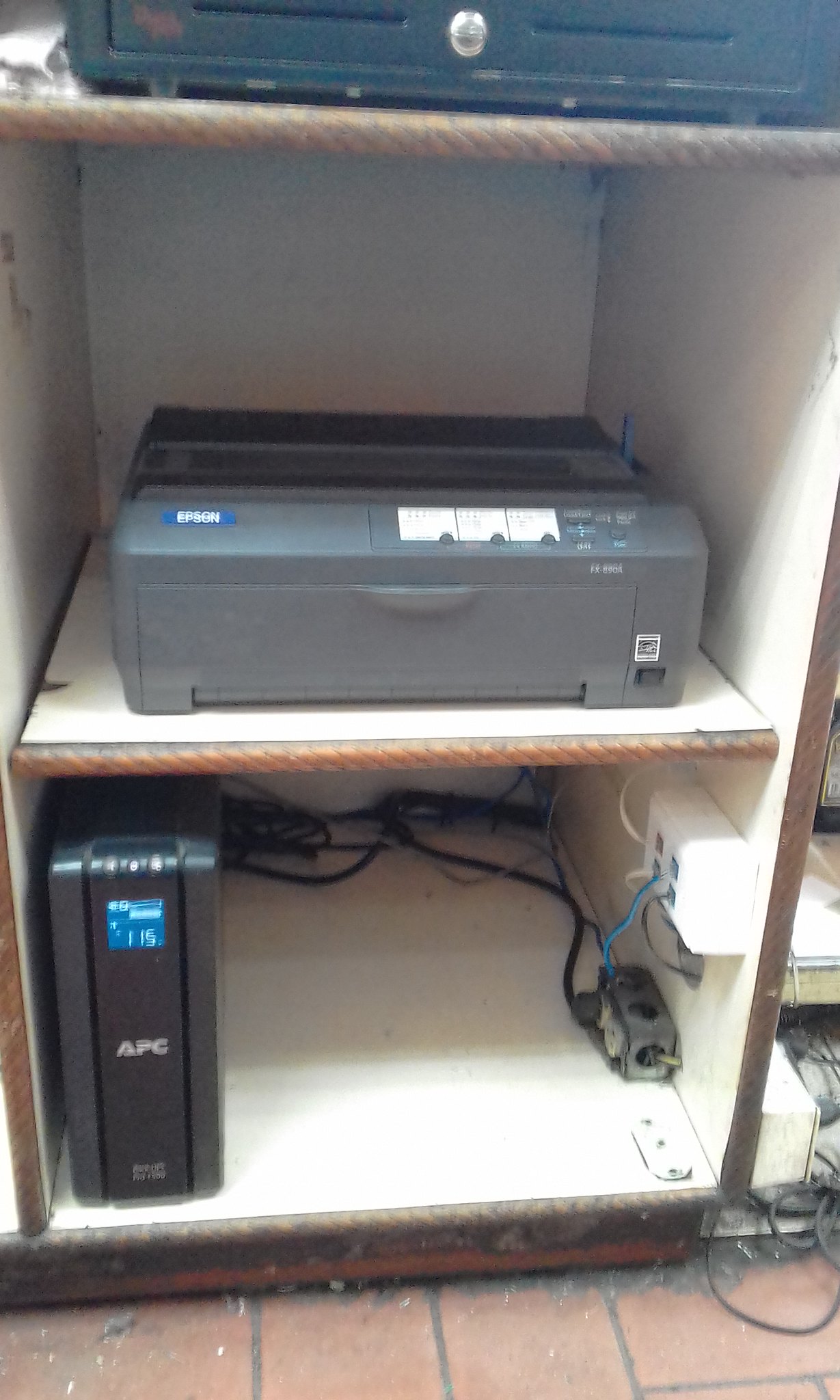This image features an open cabinet with multiple levels in a commercial setting, potentially a restaurant or store, given the dirty and debris-covered orange tile floor. The cabinet has a predominantly white structure with a brown edge. On the bottom level, there's a computer mainframe connected to a power supply, displaying electronic numbers and labeled "APC," with an assortment of black wires visible behind it. The middle shelf houses a black Epson printer. At the top, part of an indiscernible device is visible. The photo is of low quality, appearing shaky and blurred, and lacks precise cropping, making specific details harder to discern.